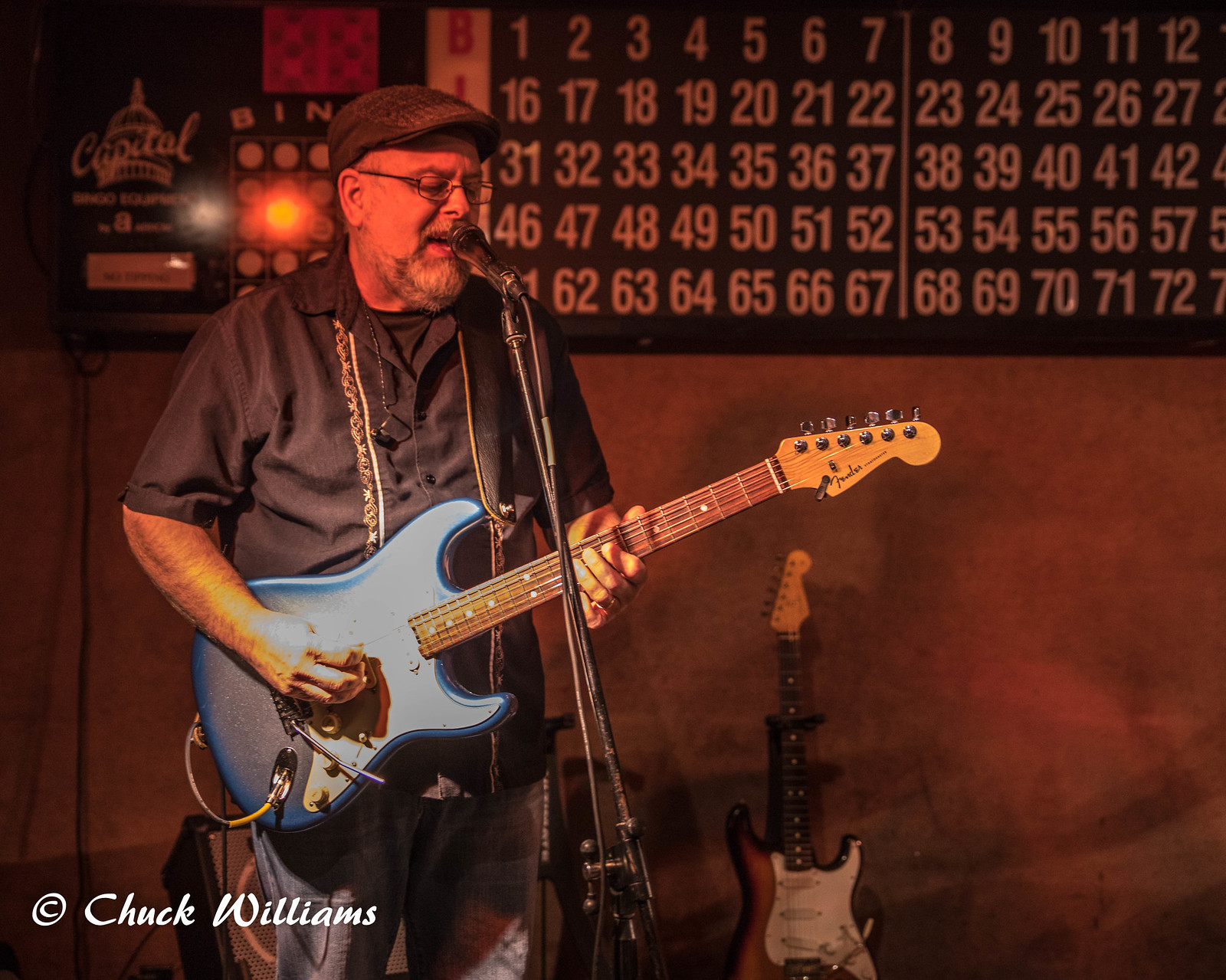In this dimly lit, reddish-orange shaded room, an older Caucasian man is captured mid-performance. He wears a painter's hat, wire-rimmed glasses, and a short-sleeved, gray button-up shirt, paired with blue jeans. His gray beard and mustache frame his face as he sings passionately into a wired microphone mounted on a metal stand. The man plays a blue Fender Stratocaster guitar.

The background features a dark wall with a white and brown electric guitar propped up against it. Above him, there's a long rectangular board; on the left side, "Bingo" is displayed in white text alongside a five-by-five grid of numbers, while the right side also shows "Bingo" in red text, partially obscured by the man. This board contains a grid of numbers ranging from 1 to 72.

In the lower left corner of the photograph, a white text watermark reads "© Chuck Williams." The overall ambiance hints at a cozy setting like a bar, where live music and bingo might share the same space.